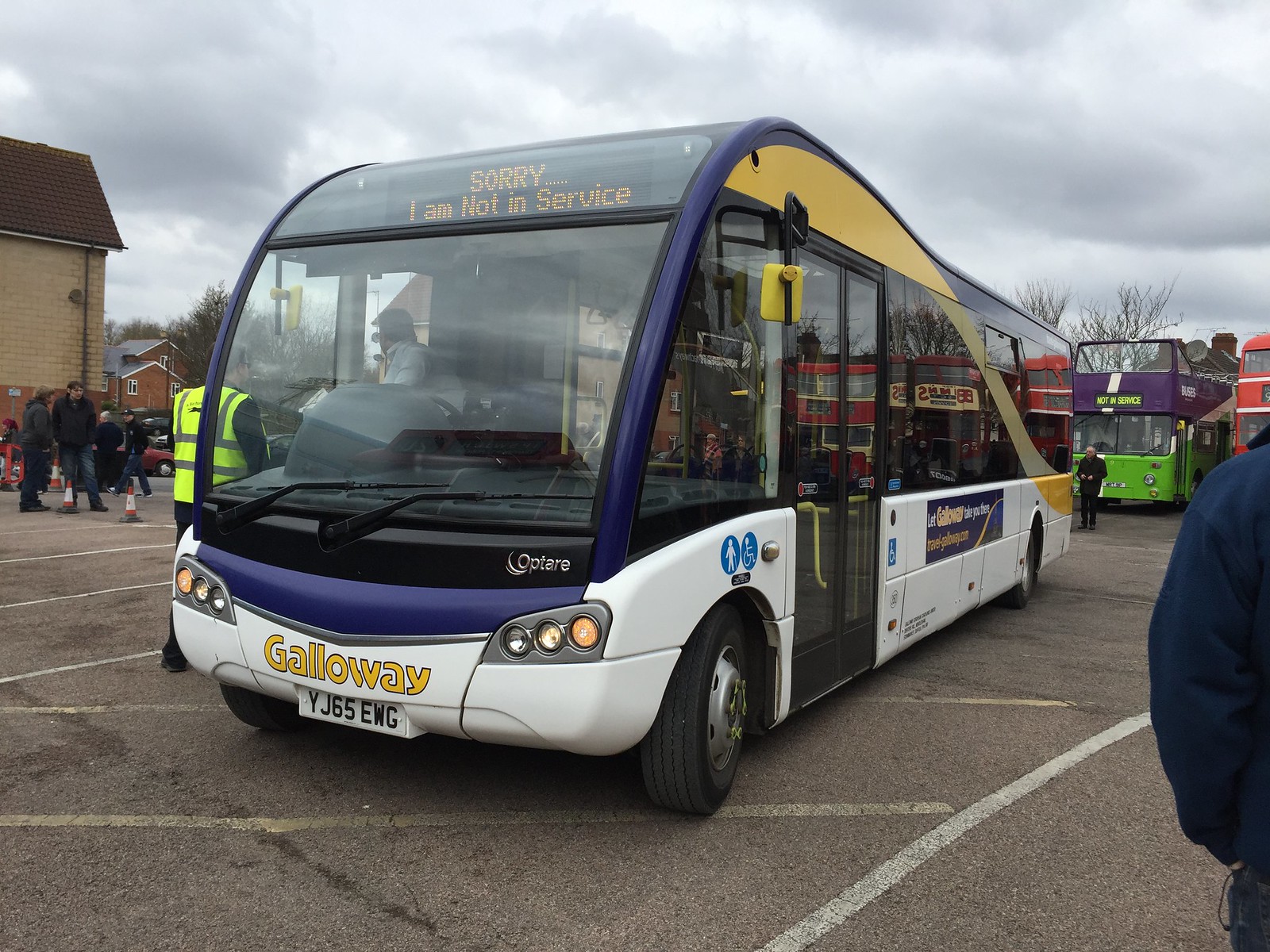This image captures a detailed scene of a modern bus parked in a parking lot, likely in the United Kingdom. The bus, labeled "Galloway" in yellow letters on the front, exhibits a white body accented with blue and yellow trim. Dominating the front view is a large, high glass windshield which arches gracefully over the top, beneath a digital sign displaying "Sorry, I am not in service" in yellow letters. The license plate reads YJ65EWG, confirming its recent model.

The photograph, taken head-on with a view of the right passenger side, reveals the presence of the bus driver inside. Also noteworthy are the sleek, modern headlights and tinted windows that add to the bus’s contemporary aesthetic. The day appears overcast, with gray clouds above, and the scene is set against an asphalt parking lot marked with lines. 

To the left of the bus, a person in a fluorescent yellow and gray safety jacket, possibly a policeman, seems to be interacting with the driver. Behind them, an old brick building with a brown roof and light brown brick walls forms part of the background. A cluster of people is seen milling about on the left, potentially waiting for transportation.

On the right side of the image, the right arm and leg of a man wearing a navy blue jacket and blue jeans can be seen, though his face is out of frame. Behind the main bus, additional buses in various colors, including a green bus with a purple top (also marked "not in service") and a partially visible red double-decker bus, line up. In the distance, the tops of trees and residential buildings with red bricks and white-trimmed roofs are visible, accentuating the setting as a busy transportation hub.